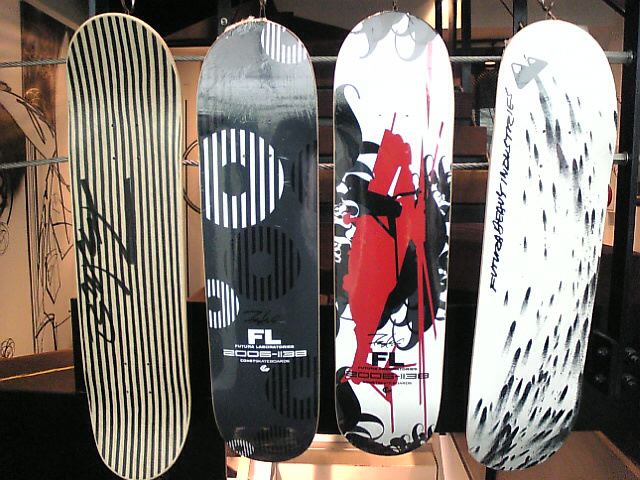The image depicts a vertical display of four boards, either snowboards or skateboards without wheels, arranged side by side with a little space in between. Each board showcases a unique design, with the first on the left featuring black and white vertical stripes and some center lettering. The second board has a black background adorned with white striped circles at the top, center, and bottom, and includes the letters "FL" with additional unreadable text, possibly including the numbers "2006-138." This board appears to have no bindings and is facing the camera, seeming to float against a brownish background. The third board, next to it, presents a splattered pattern of white, black, and red, also bearing the "FL" initials and indiscernible text below them. The final board on the right is primarily white with black splashes and has some unreadable script at the top. All four are oriented upright, contributing to an overall artistic and visually captivating arrangement set against a mostly brown backdrop.